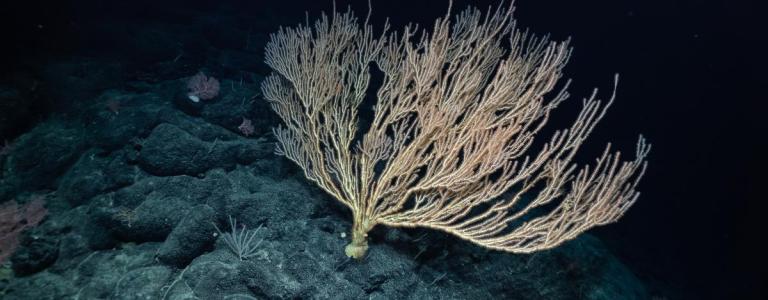This is a detailed underwater photograph capturing a striking ocean landscape. The image, much wider than it is tall, features a dark, almost black background, highlighting the stark contrast of its illuminated subject. Dominating the center is a wide, beige sea plant that resembles an intricate, spindly structure, akin to a tiny tree trunk with branches that spread out delicately. This central piece appears light brown or yellowish, showcasing a fascinating, almost velvety texture.

The plant grows from a rugged, bumpy rock formation on the ocean floor, which is slightly visible to the left of the image with discernible textures and minor growths. The rock underneath appears dark greenish-blue, adding to the textured, layered composition. Interestingly, some purple sea creatures are also present, clinging to this rock, providing a splash of color amidst the darkness.

The top left of the image fades into deep black, further emphasizing the isolation and prominence of the central sea plant. This photograph, captured near the ocean's bottom, beautifully contrasts the intricate coral formation against the void-like backdrop, making the underwater flora the undeniable focal point.